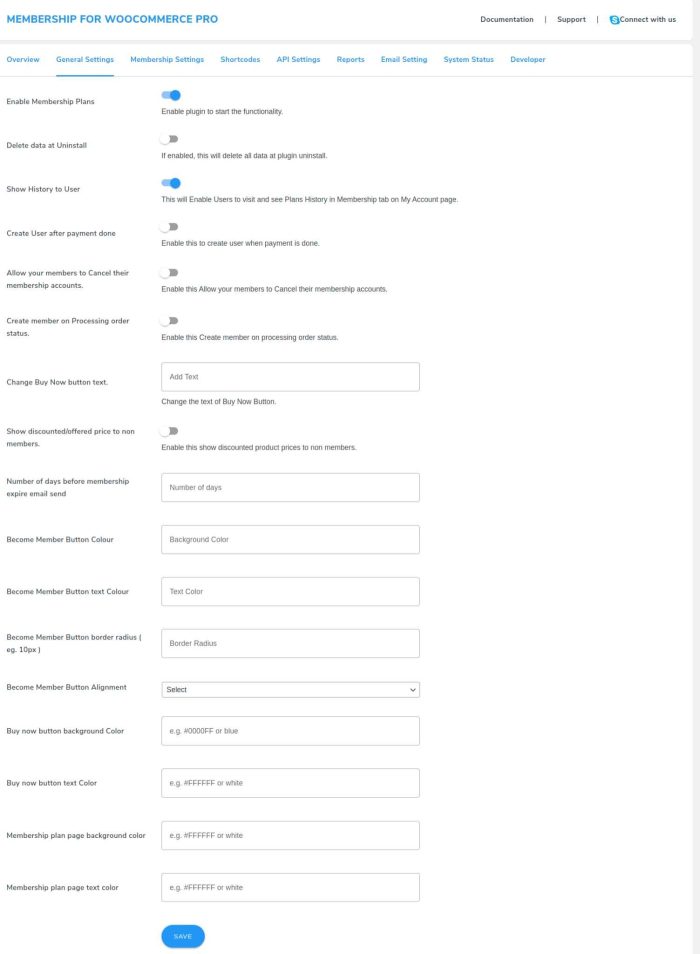### Detailed Caption for the Web Page Screenshot:

This screenshot captures a blurry view of a webpage with a white background, making the text difficult to read. Despite the blurriness, several key elements can be discerned:

- **Header:**
  - The header features text in blue font reading **"Membership for WoodCommerce Pro"**.
  - To the right of the main header text, in black font, are several links separated by vertical black bars: **"Documentation"**, **"Support"**, and **"Connect with Us"**.

- **Navigation Bar:**
  - Directly below the header is a gray horizontal bar serving as a secondary navigation area.
  - Below this, a series of options in blue font are listed, each representing different sections of the settings menu:
    - **Overview**
    - **General Settings** (this option is selected, underlined in black)
    - **Membership Settings**
    - **Shortcodes**
    - **API Settings**
    - **Report**
    - **Email Settings**
    - **System Status**
    - **Developer**

- **Content Area:**
  - Under the **General Settings** section, the first option presented is titled **"Enable Membership Plans"** in black font.
  - This is followed by a list of other settings options, each in black font:
    - **"Delete Data at Uninstall"**
    - **"Show History to User"**
    - **"Create User After Payment Done"**
    - **"Allow Your Members to Cancel Their Membership Account"**
    - **"Create Member on Processing Order Status"**
    - **"Change Buy Now Button Text"**
    - **"Show Discounted Offered Price to Non-Members"**
    - **"Number of Days Before Memberships Expire Email Send"**

The overall page structure suggests a user interface designed for managing membership options within the WoodCommerce Pro platform, with a clear layout demarcating settings and configuration options.